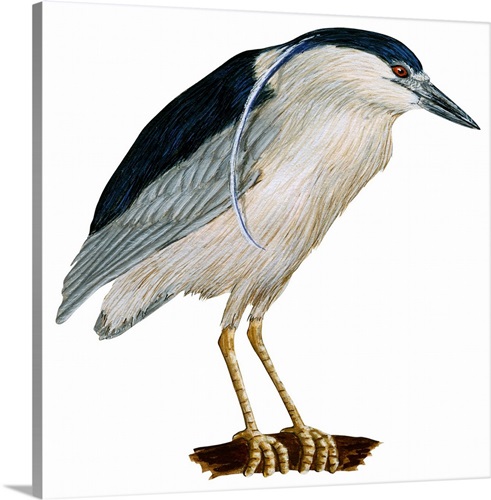This image features a detailed painting of a bird with a bordered frame, suggesting it is a product image available for purchase. The bird in the painting has distinctive features, including a white belly with white feathers extending up its front, around its cheeks, and neck. It has striking long blue plumage that curls from the top of its head, resembling a ponytail. The bird's head and back are adorned with a dark blue color, transitioning to lighter blue on the edges of its wings. It has a long, dark beak and noticeably long, slender yellow legs, indicative of its non-waterbird classification given the absence of webbing on its feet. The bird appears to be slightly bending over or arching its back, adding dynamic posture to the artwork. The painting is set against a white background, emphasizing the bird's detailed and vibrant plumage.